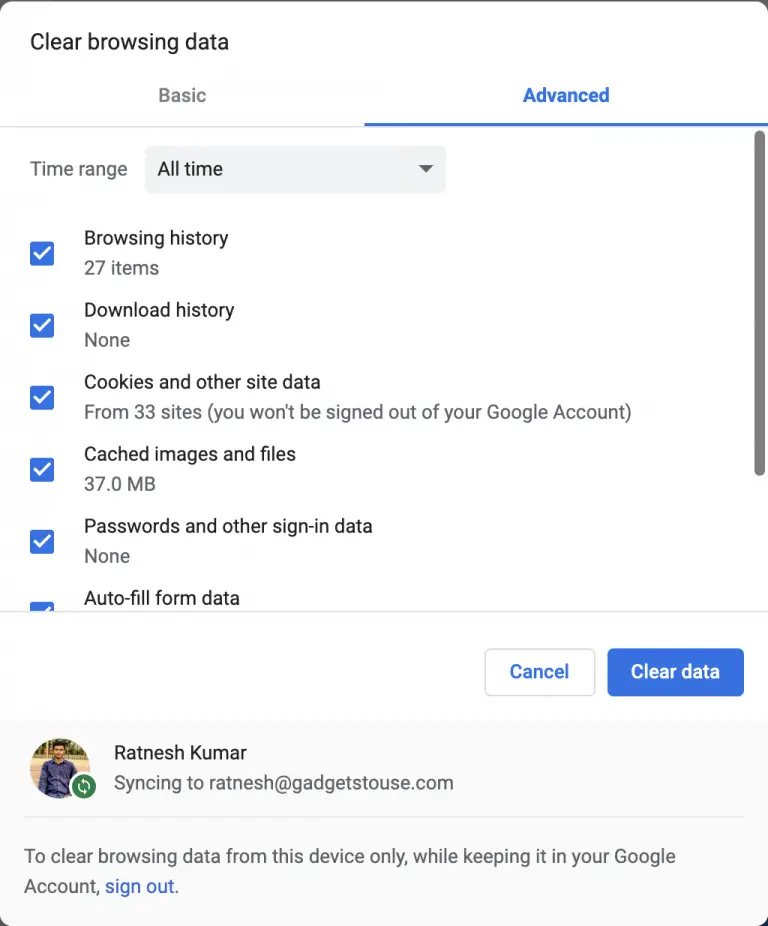This image is a screenshot of a website interface for clearing browsing data. At the top, there's a thin horizontal line. On the left side, the phrase "Clear Browsing Data" is prominent, with a capitalized "C". Below the header, the interface is presented on a white background. On the left, the options "Basic" and "Advanced" are displayed, with "Advanced" in blue text, capitalized, and underlined.

Underneath, there is a section labeled "Time Range" on the left side, accompanied by a drop-down menu showing "All Time" with a capital "A". Below this, a list of items each with corresponding checkboxes is shown, all of which are checked off in blue with a white check mark.

The items listed are as follows:
- Browsing History: 27 items
- Download History: none
- Cookies and other site data: from 33 sites
- Cached Images and Files: 37.0 MB
- Passwords and other sign-in data: none
- Autofill form data (partially obscured)

At the bottom of the interface, there are two options: "Cancel" and "Clear Data". "Clear Data" is highlighted with a blue background and white text. Further down, a user profile is displayed with a circular user picture, the name "Ratnesh Kumar", and the email address "singingtoratnesh@gadgetshouse.com".